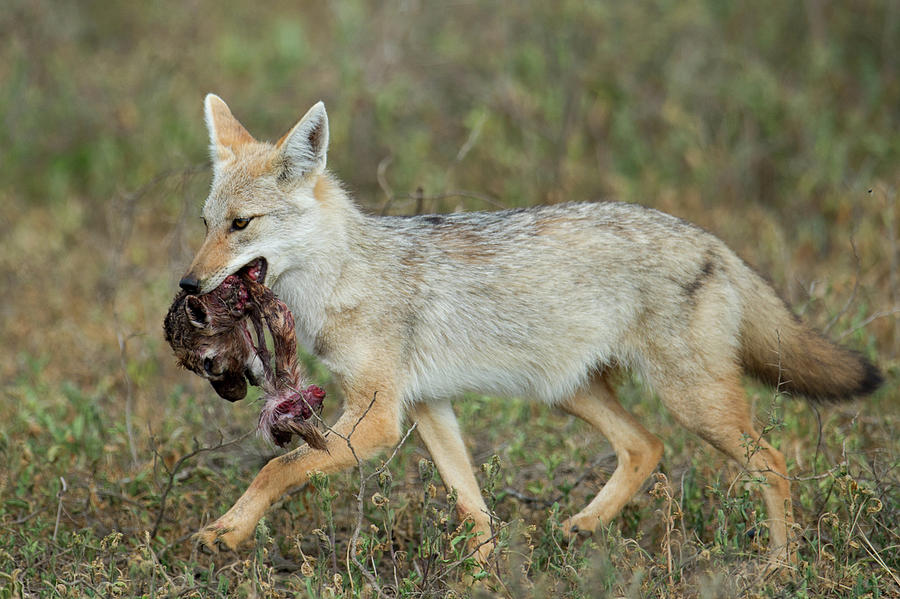The image depicts a young, light gray coyote proudly trotting through a dry, mostly brown field, carrying a piece of carnage—possibly a bird or another small animal—in its mouth. The coyote’s body displays a mixture of colors: light gray fur with spots of tan and some black tipping, particularly on its bushy tail and long legs. Its snout, ears, and legs are tan, and the tail is tipped in black. The animal's gait is peppy and lively, and it appears to be heading towards the left-hand side of the image. The background is blurred, keeping the focus on the coyote, which seems very excited about its catch. The overall scene suggests a natural outdoor setting without much greenery, dominated by dried grass and weeds.